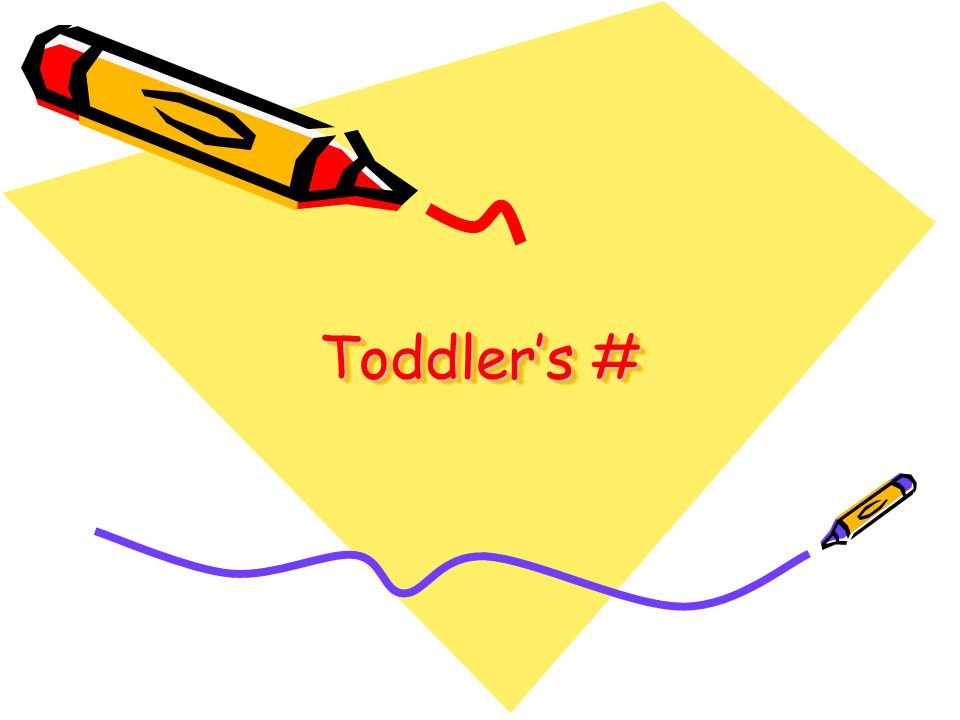The image is a detailed computer-generated drawing set against a white background. The central element is a large, slightly warped yellow trapezoidal sheet of paper, appearing diagonal and seemingly floating in mid-air. Dominating the upper left section of this paper is a large red crayon, identifiable by its dual red tips and yellow label. The crayon draws a squiggly red line atop the paper. Beneath this, in bold red font, is the word "toddlers" followed by a hashtag symbol. Towards the lower section of the image, spanning from the white background onto the bottom corner of the sheet of paper, is a blue squiggly line connected to a smaller purple crayon on the right side of the image. This crayon also features two blue tips and a yellow label, echoing the design of the larger red crayon.